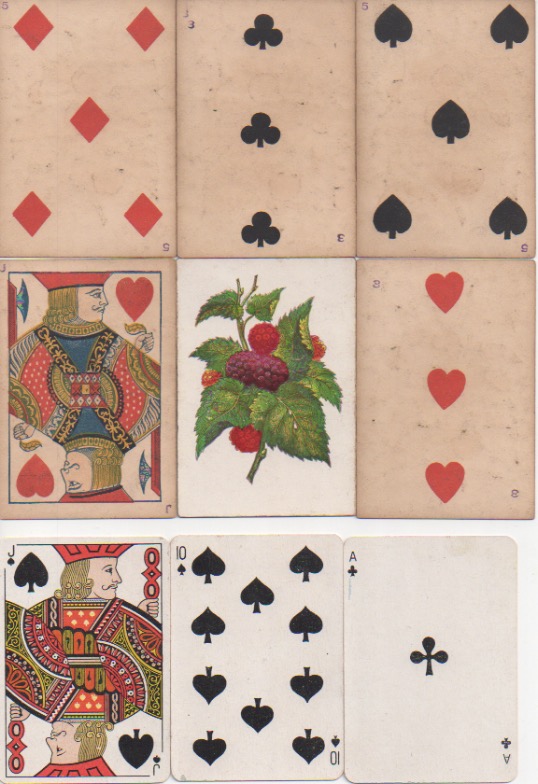This poster-sized image depicts a photograph of nine vintage playing cards arranged in three evenly spaced rows of three against a white background. The cards, which appear old and weathered, vary in color from dark red to tan. In the top row, from left to right, are the 5 of diamonds, the 3 of clubs, and the 5 of spades. The second row features a jack of hearts, a card showing a trio of red and purple berries with leaves on the back facing up, and a 3 of hearts. The bottom row consists of a jack of spades, a 10 of spades, and an ace of clubs. The overall presentation suggests a vintage aesthetic, with the cards exhibiting signs of aging, such as graying or sun-bleached pink hues.